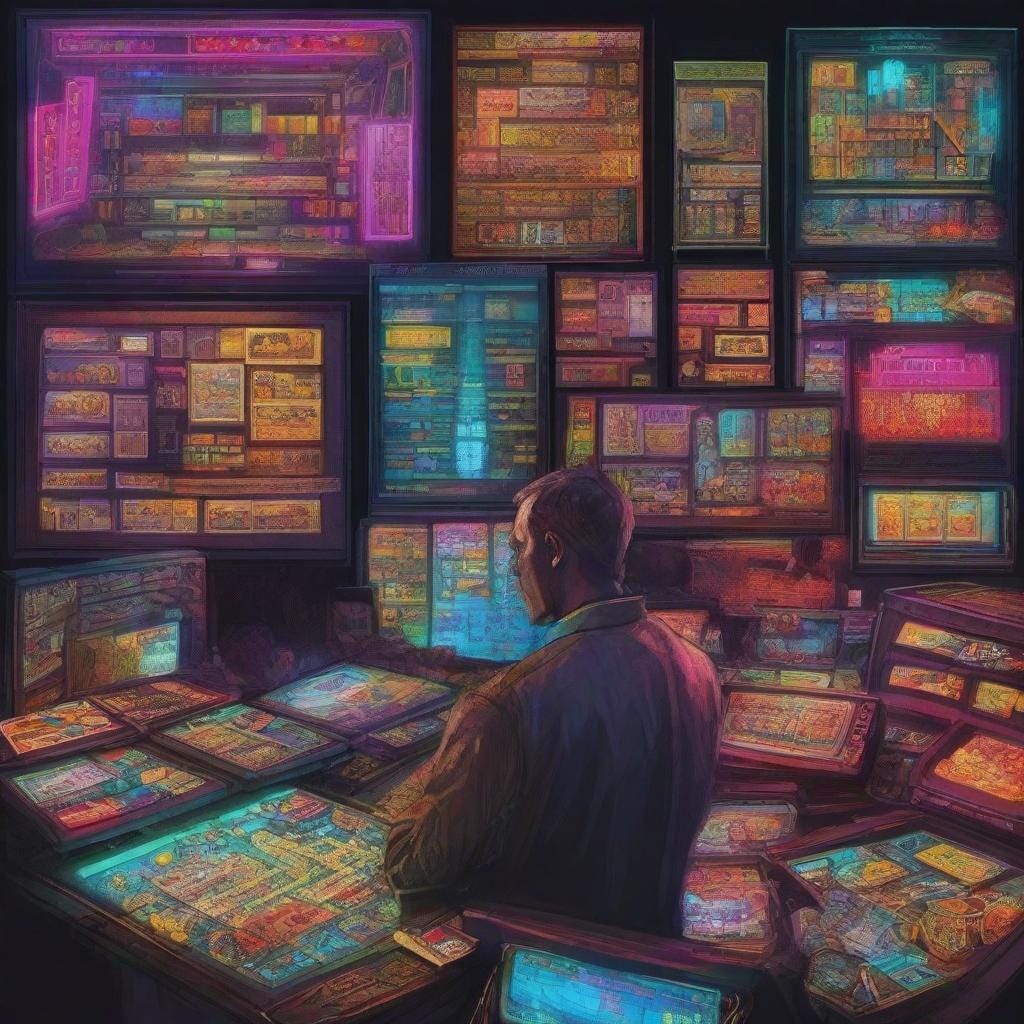In the illustrated image, a man with short hair, dressed in a business-like shirt, is sitting at a table, immersed in a vibrant, neon-colored environment. Surrounding him on the table and mounted on shelves are numerous frames and screens, each containing abstract elements. These frames, filled with neon hues of pink, blue, green, yellow, and purple, vary in size and shape, creating a visually striking collage. The man appears to be in a setting that could be a control center or library, deeply studying the contents of these frames. Some frames resemble maps or tickets, though the details within them are elusive, adding to the abstract nature of the scene. The illustrations are highly detailed and colorful, with outlined squares and blocks of color captivating the observer’s attention, giving a sense of endless information and artistic complexity.